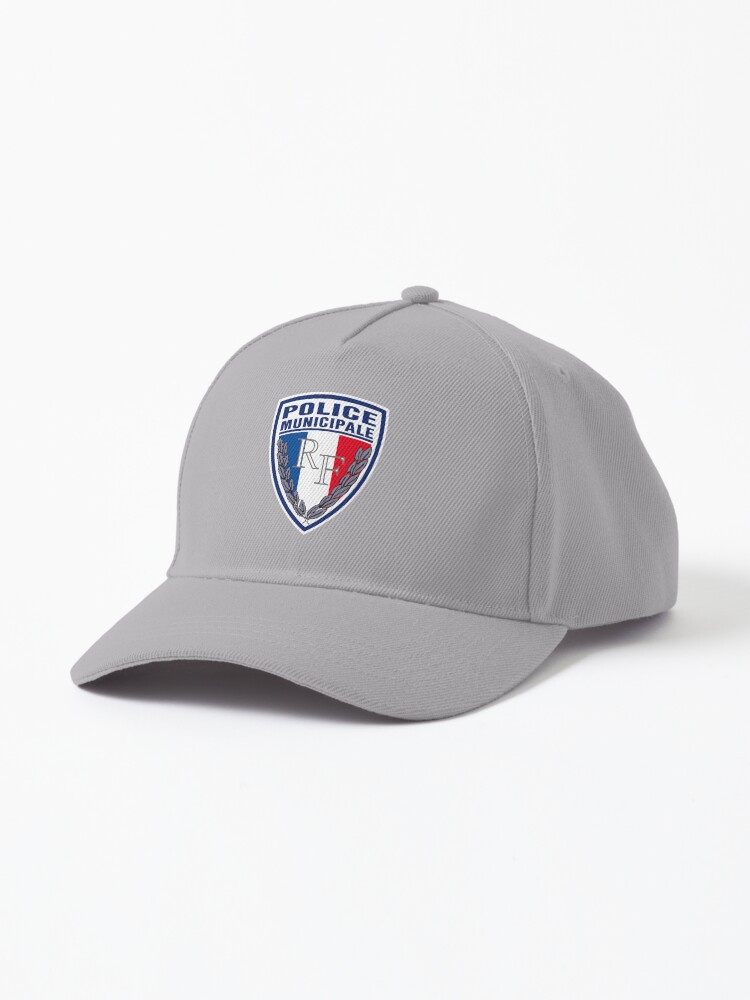The image features a medium gray fabric baseball cap set against a white background. Prominently displayed on the front center of the cap is a shield-shaped emblem resembling a police badge. The badge has a white background with a thin dark blue border. At the top of the shield, in dark blue text, are the words "Police Municipale." Below this text, the bottom half of the shield is vertically divided into three sections: blue on the left, white in the middle, and red on the right. Centered over these sections are the initials "RF," and flanking the shield are two gray wreath leaves that extend from the bottom center to the top left and top right edges of the emblem.